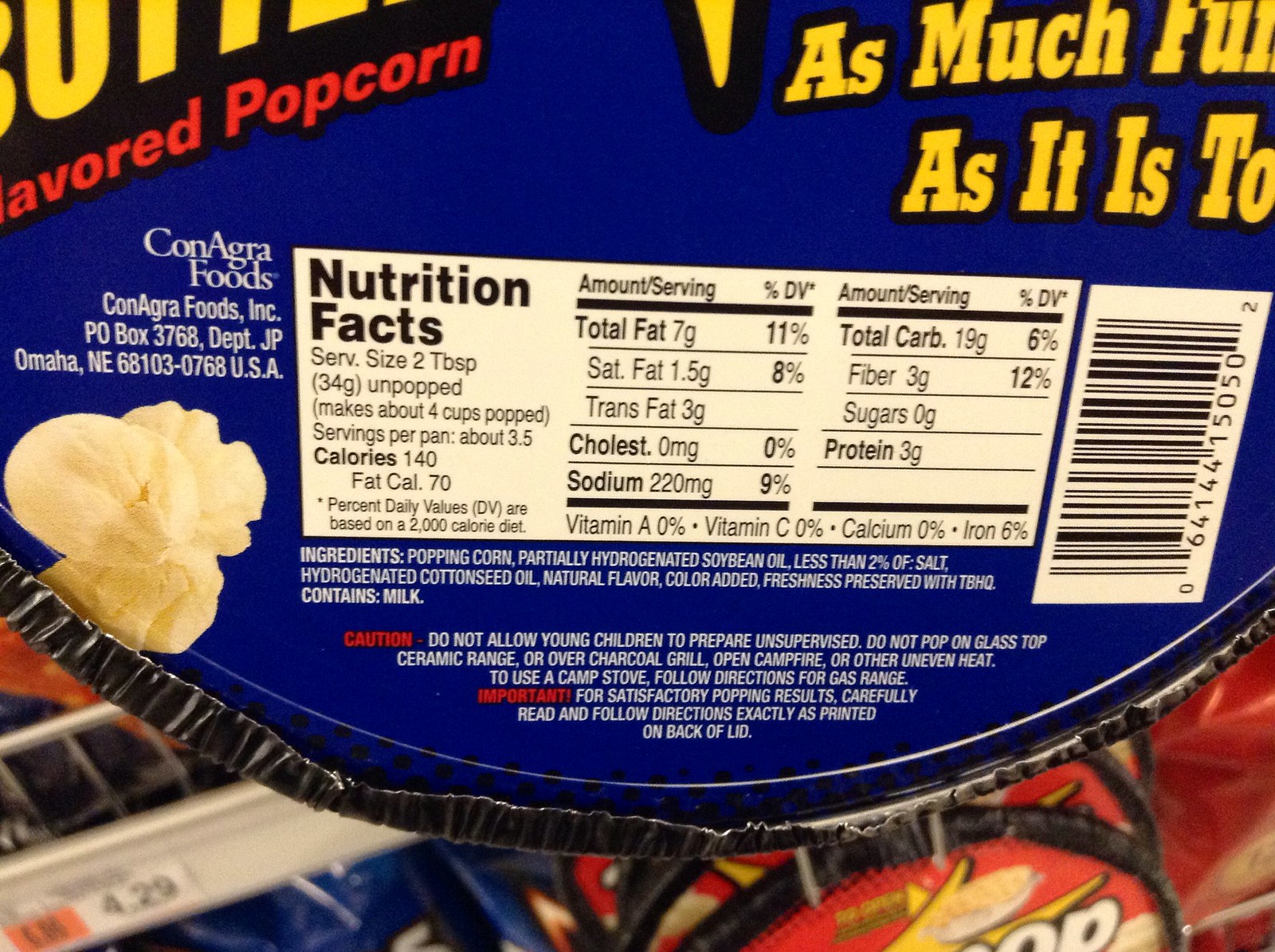This detailed image showcases a box of Jiffy Pop popcorn, prominently featuring the nutritional label and several key elements. The packaging is designed with a dark royal blue background and contains text in both red and yellow colors that spell out parts of words like "B-U" and "A-B-O-R-E-D". Manufactured by ConAgra Foods, Inc., located in Omaha, Nebraska, the popcorn is designed to be popped over a flame or stove because it's encased in an aluminum foil pan, which is clearly shown to be unsuitable for microwave use. The nutritional facts are clearly outlined: a serving size is 2 tablespoons (approximately 34 grams unpopped), and each pan makes about 4 cups of popped popcorn, with around 3.5 servings per pan. Each serving contains 140 calories (70 of which are from fat), 7 grams of total fat (11% of DV), 1.5 grams of saturated fat (8% of DV), 3 grams of trans fat, 220 milligrams of sodium (9% of DV), 19 grams of carbohydrates (6% of DV including 3 grams of fiber), zero sugars, and 3 grams of protein. The ingredients listed include popping corn, partially hydrogenated soybean oil, less than 2% salt, hydrogenated cottonseed oil, natural flavor, artificial color, and a preservative (TBHQ) for freshness, with a warning that the product contains milk. There are specific cautions and instructions advising against letting young children prepare the popcorn unsupervised and not to pop it on glass, ceramic ranges, or over open campfires. The price tag visible in the image shows $4.29, and a barcode numbered 0-641-441-5050-2 is also present. The box's instructions recommend careful adherence to ensure satisfactory popping results.